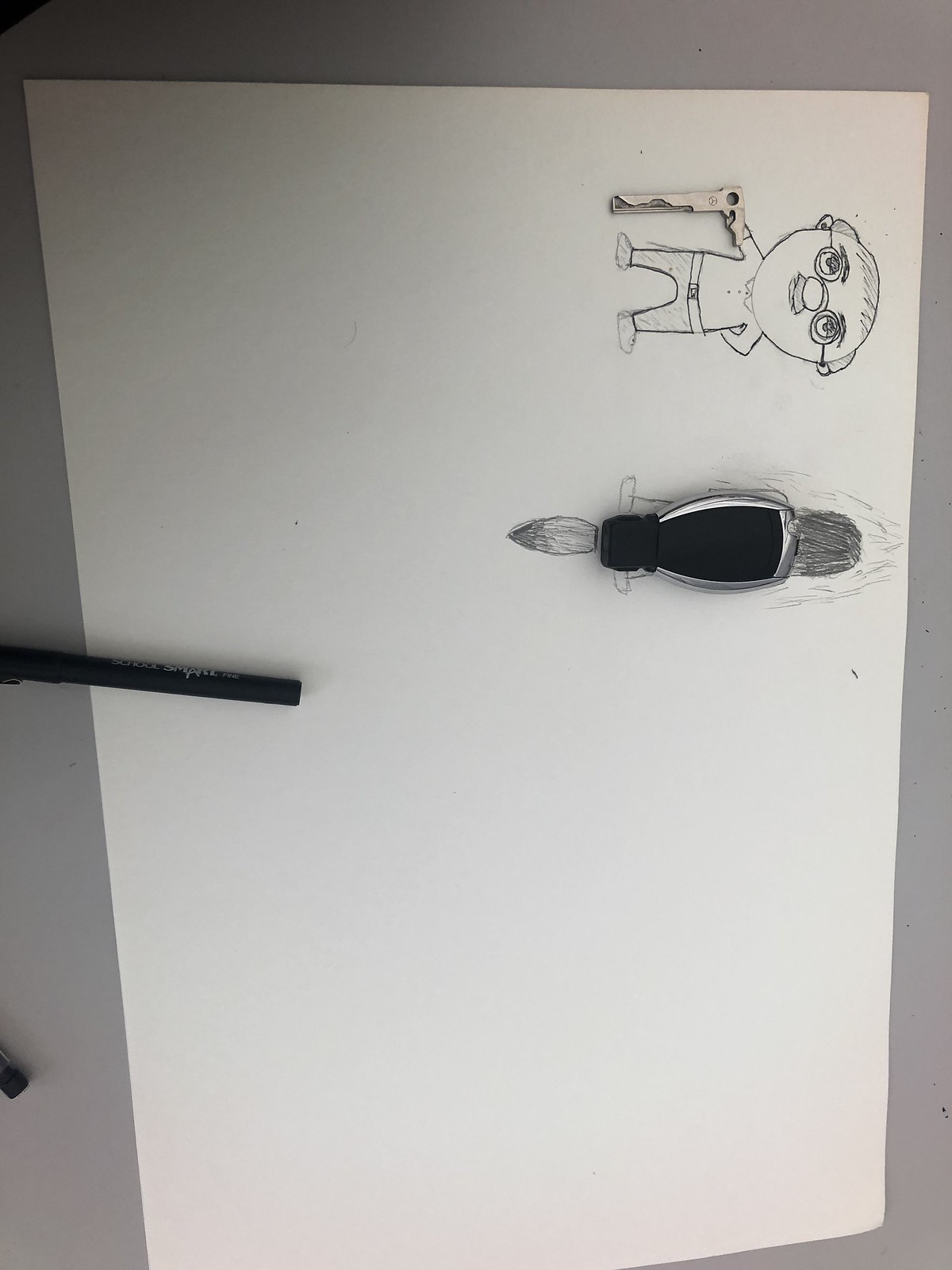The image depicts an art piece on a sheet of white sketching paper, captured with the drawing oriented sideways, indicating either the paper or the camera was rotated incorrectly. At the top right of the sheet, there is a detailed pencil sketch of an elderly man. The man, wearing glasses and holding a cane, is rendered intricately, with careful attention to his facial features and attire. Notably, the cane appears to be a three-dimensional element, potentially made from a metallic material and affixed to the paper, adding a unique mixed-media dimension to the drawing. Adjacent to the elderly man, there is a mysterious black object that might represent a paintbrush, though its exact nature is unclear. The illustration is set against a plain backdrop with no accompanying text.